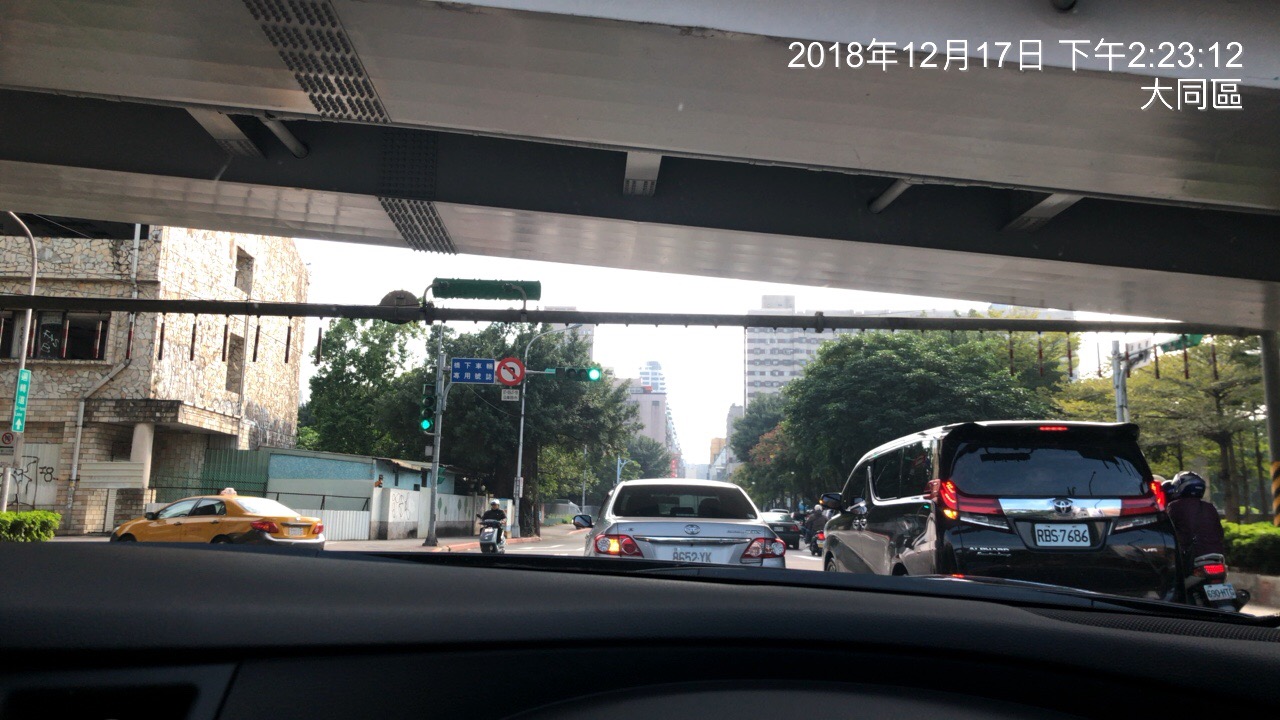A wide-angle dash camera view captures a bustling urban street scene underneath an overpass. Several cars are lined up at a stoplight, which has just turned green, allowing the vehicles to start moving forward. Directly in front of the camera is a small silver car, while to its left is a large black minivan, and to the right of the minivan, a motorcycle can be seen. A taxi is visible making a left turn in the background, near the center-left of the photo. Overhead, the underside of the bridge is visible, framing the scene above the vehicles. Two stoplights are discernible in the background: one on a taller pole to the left and another on a shorter pole directly beside it. At the top right corner of the image, the date "2018/12/17" and the time are displayed, accompanied by several Chinese characters. The dashboard of the car from which the photo is taken is also partially visible at the bottom of the image, showing it to be black.